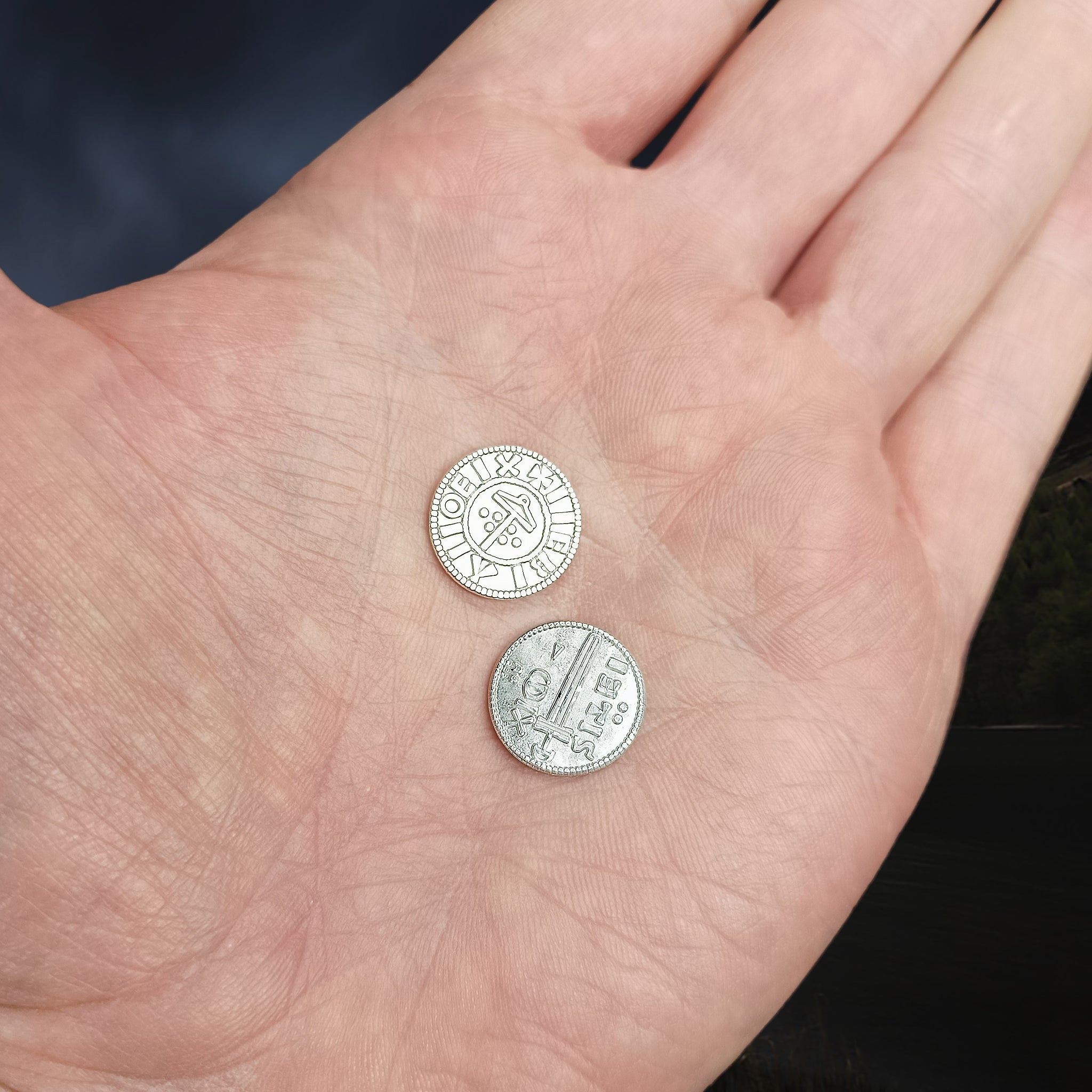The image is a close-up, high-detail photo of an open palm belonging to a white person with a light, slightly reddish-toned skin, indicative of cold. The hand is outstretched against a dark, gray and black background that highlights its features. Nestled in the center are two small, silver-colored coins, slightly smaller than a dime. These coins, likely ancient, display different designs, possibly hieroglyphics or other intricate symbols, suggesting their foreign origin. The coin positioned higher in the image appears cleaner and in better condition than the tarnished, dirtier one below it. The hand is held closely together, with no gaps between the fingers, enhancing the focus on the detailed textures of the coins and the hand.